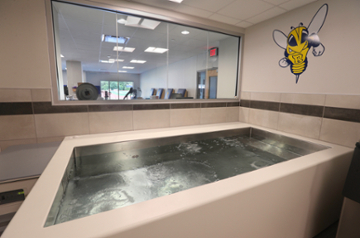This image depicts a recovery ice bath or jacuzzi in a sports training center, identifiable by its large, square stainless steel bathtub filled with clear water. The room's decor is notable for its pink walls accented by a brown stripe about halfway up. Above the tub on the right wall, there's a prominent yellow jacket or hornet logo, characterized by an "R" on its chest, in striking yellow and black colors. Adjacent to this area, a glass window provides a view into an adjacent room that appears to be a gym or fitness facility. This space is equipped with workout equipment, including barbells and seating areas, and features white walls. Through the glass, one can also see an exit door marked by a red exit sign, as well as a hint of the outside world with visible green trees and bright daylight. The gym also showcases reflective ceiling tiles and sunroof glass, adding to the room's bright, airy ambiance. The entire setting is finished with tile, complementing the facility's functional yet aesthetically cohesive design.